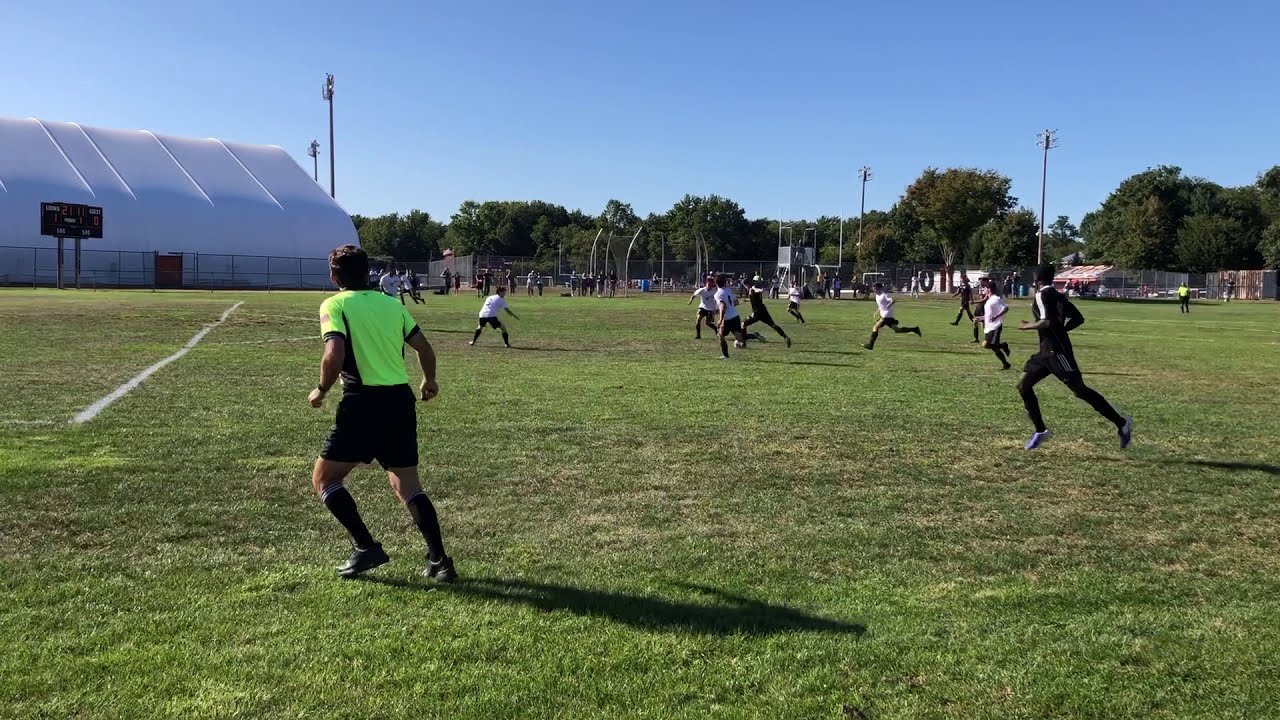The image captures an outdoor soccer match on a grass field with mixed patches of green and dry yellowed grass. The field is outlined with white lines and surrounded by a silver gate. The players, appearing to be young males aged 17-25, are divided into two teams wearing black and white uniforms. The main action is centered on the left side of the image, where three players in white uniforms are intercepting a player in black who has the ball, while more players from both teams close in. A referee dressed in a neon yellow-green shirt with black sides, black shorts, knee-high black socks with white lines, and black shoes is seen running towards the active play. He is looking at the players and the ball with his back to the camera. 

In the background, a large white pavilion-like structure and a black scoreboard, showing a score of 1-0 and a time of 21:11, are visible. Surrounding the field, there are green trees and tall stadium lights on silver poles. The sky is a bright, clear blue with no clouds, providing a sunny atmosphere. An audience is also present, watching the ongoing soccer match.